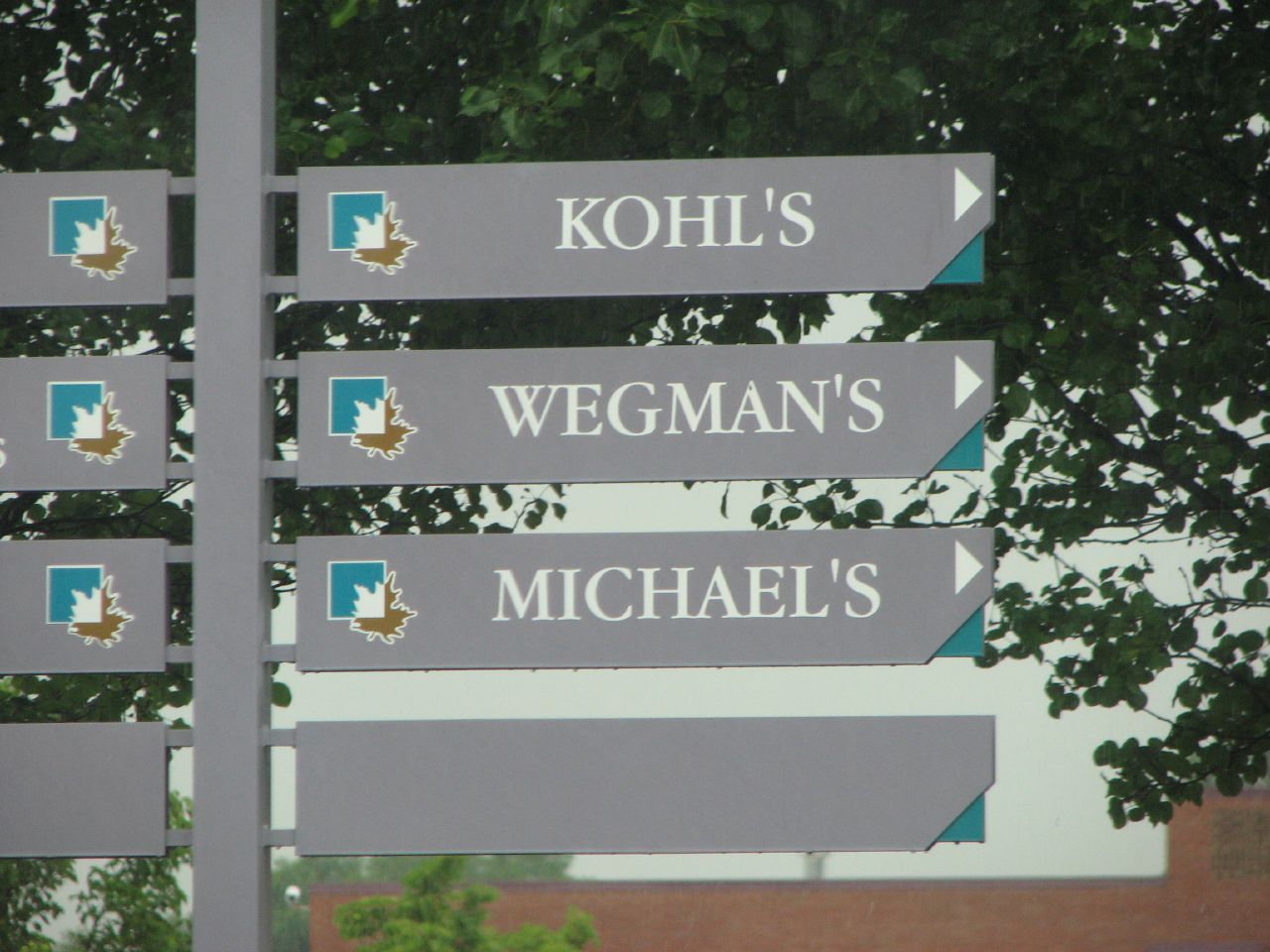This photograph, taken in a somewhat dimly-lit outdoor setting, depicts a series of directional signs lined up on a gray metal post, suggestive of a shopping center or mall parking lot. The image, which is wider than it is tall, emphasizes the signage against a backdrop of greenery and what appears to be a building in the distance. 

Each sign consists of a teal square with a brown maple leaf overlapping logo, followed by an arrow indicating direction. At the topmost position on the right side, a sign points to "Kohl's" with a white arrow leading to the right. Below that, another sign directs towards "Wegmans," followed by a sign for "Michaels," with the bottommost sign left blank. The signs each have a teal backing visible behind them, which contrasts with the gray metal post.

The post's bottom right portion is slightly cut off in the photo, revealing more of the teal background beneath the signs. The overall scene is framed by greenery with a building partially visible behind it, contributing to the commercial and organized feel of the location.